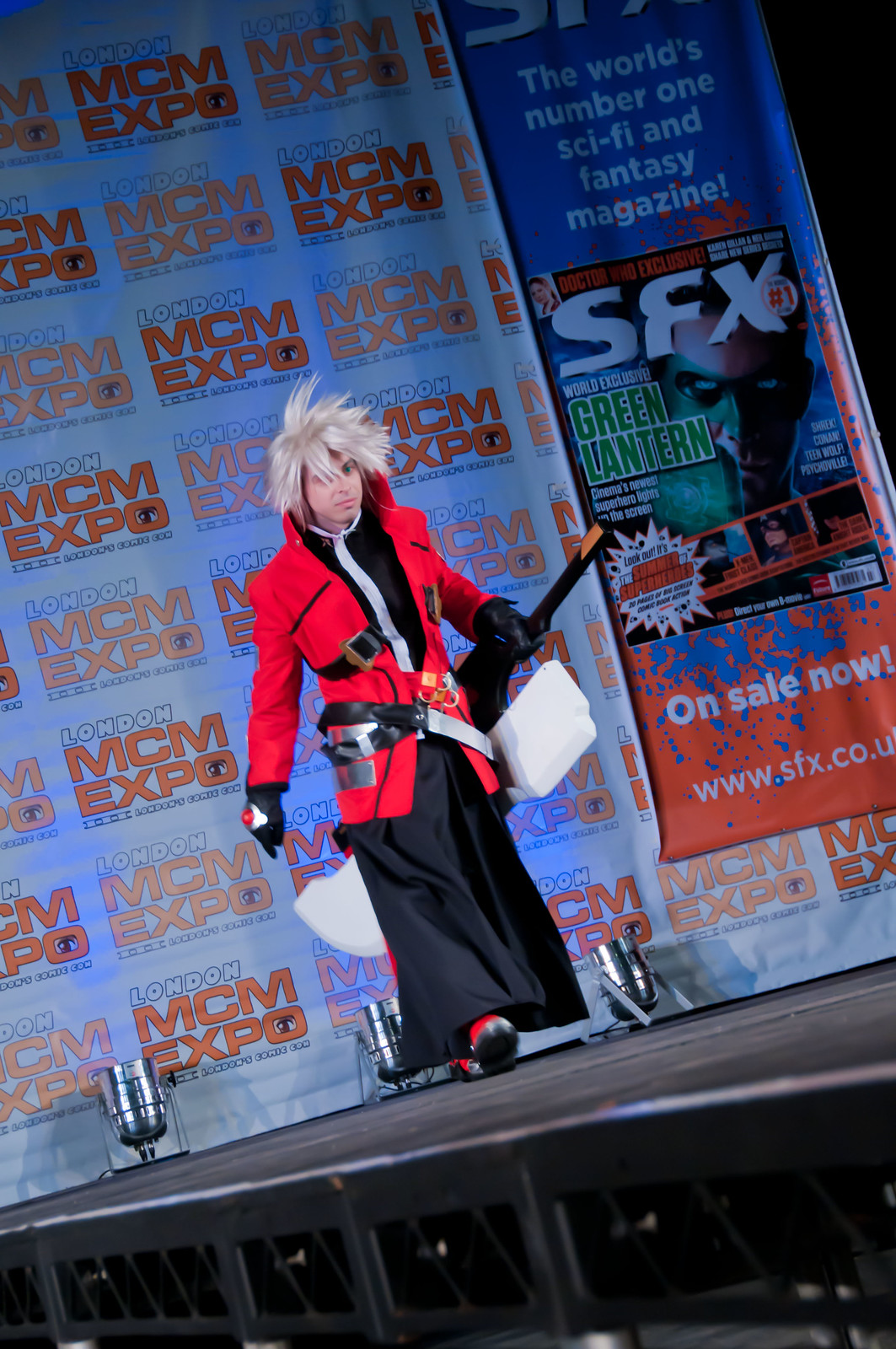The image depicts a male cosplayer walking across a slightly angled, black, raised stage, adding a dynamic feel. He stands out with his striking light blonde, spiky wig that points forward and to the side. Adorned in a red jacket layered over a black and white shirt, and long, wide-legged black pants, his ensemble is completed with bright red shoes featuring black soles. He accessorizes with black gloves, one of which has a red dot on top. A heavy belt at his waist supports a white sword sheath, and he wields a black anime sword in his hand. Behind him, three silver spotlights aim dimly toward a large, blue backdrop, which prominently displays "MCM Expo London" in orange and red lettering along with "SFX Greenland" and a callout to a magazine cover with cinema-related headlines.